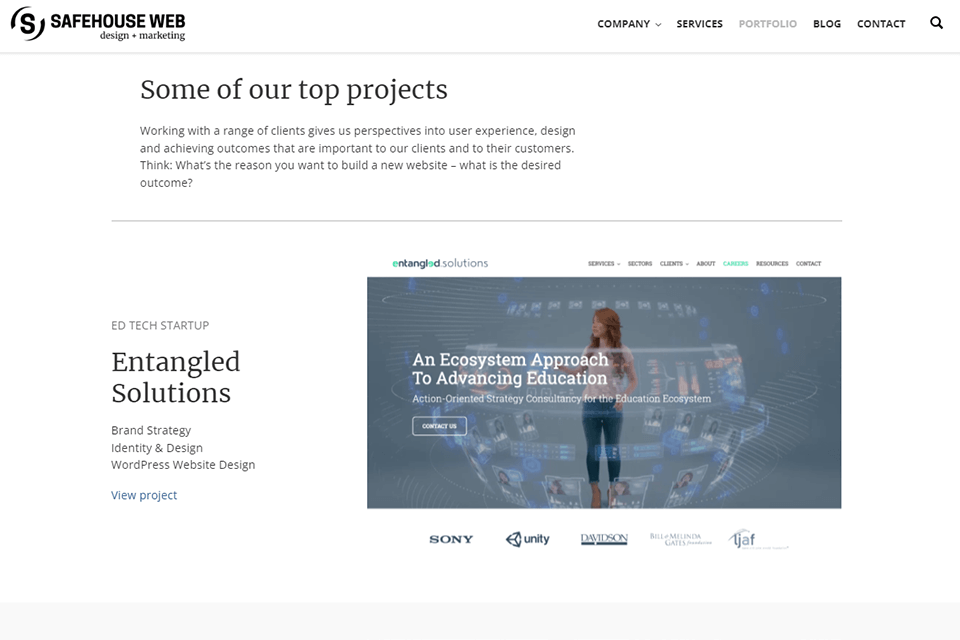The landing page of Safehouse Web Design and Marketing, highlighted in this image, exemplifies their expertise as a premier web design and marketing company. Dominating the page is a dynamic visual of a woman engaging with a futuristic digital display, encapsulating the innovative essence of their brand. The Safehouse Web logo and a well-organized navigation menu reside at the top, offering quick access to sections such as Company Information, Services, Portfolio, Blog, and Contact.

Prominently featured on the page are details of their top-tier projects, notably their collaborations with Entangled Solutions and a notable ed tech startup. These projects span across brand strategy, identity and design, and WordPress website development, underscoring their comprehensive service offerings.

The page is meticulously designed to emphasize exceptional user experience, cutting-edge design, and significant customer outcomes. Partnerships with industry giants such as Sony and Unity are acknowledged, showcasing their credibility and collaborative prowess.

Interactive elements include a blue hyperlink allowing users to view individual projects in detail, a search bar to navigate the website efficiently, and a drop-down menu under the Company tab that potentially reveals additional partner companies or related services offered. This landing page is a testament to Safehouse Web Design and Marketing's commitment to innovation and excellence in the digital space.